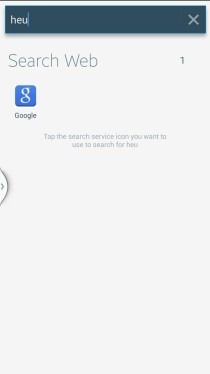In this image, we observe a minimalistic interface predominantly featuring a white background. At the top of the image, there is a search box with partially typed text "H-E-U," indicating an incomplete search query. To the right of this search field is a cancel button, represented by an 'X.' Below the search box, the iconic Google app is displayed in blue. Throughout the image, instructional text reads, "Type the search service icon you want to use to search for H-E-U." The top portion of the image is shaded grey, while the rest of the background remains white. Overall, the image is characterized by a clean, uncluttered design with no other elements present.